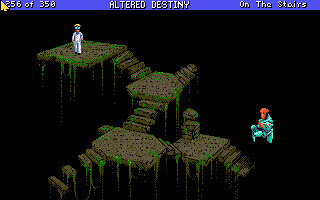The image is a screen capture from an old video game displayed on a computer monitor. Dominating the screen is a vibrant blue bar across the center, prominently featuring the title "Altered Destiny." In the top right corner, additional text reads "On the Stairs." The computer screen itself is predominantly black, serving as a dramatic backdrop for the in-game scenery.

The game environment presents a series of moss-colored stairs, beginning in the bottom left corner and ascending in a staggered fashion across multiple landings. These stairs wind through the image, creating a labyrinthine pathway that culminates at the top landing. The main video game character, situated on this uppermost platform, is depicted in a white shirt and pants, and accessorized with glasses.

Interestingly, a secondary character is positioned to the right, seemingly floating in the black void. This figure is dressed in blue attire and wears a striking red helmet, adding a splash of vibrant color and intrigue to the stark, eerie setting.